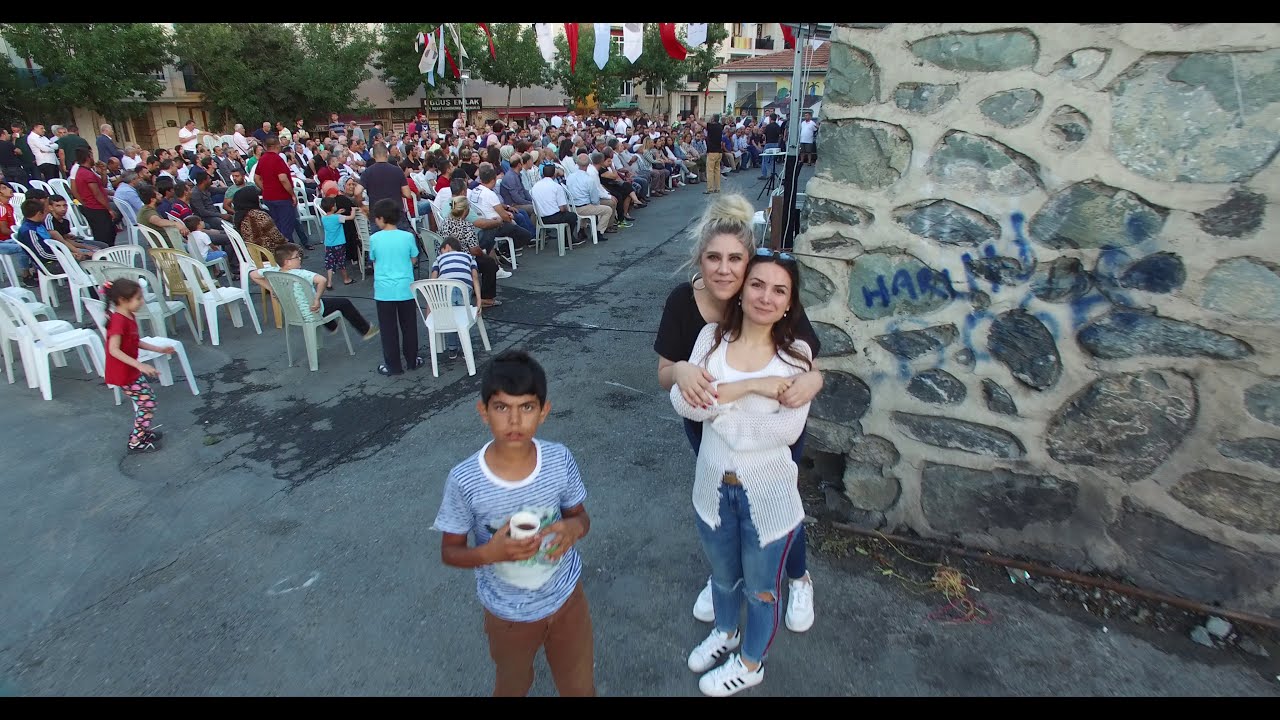In this image, set within a rectangular frame with black bands across the top and bottom, three central figures stand prominently on a dark gray paved surface at an outdoor event. On the left stands a small boy with dark hair and brown skin, dressed in a blue and white striped T-shirt and brown pants, holding a white cup filled with dark liquid in front of his chest and looking up at the camera with a puzzled expression. On the right, one woman with long brown hair, wearing a white top, blue jeans with a red stripe down the side, and white sneakers, stands in the front. She has sunglasses perched on her head and is holding the hands of another woman standing directly behind her. The woman behind has blonde hair, wears a black top, and has large round earrings. 

To their right is a high stone wall, with shades of gray and beige and tan-colored grout lines. Some blue graffiti is visible on the wall. The background behind the group is filled with white plastic chairs occupied by a diverse crowd, suggesting a large gathering or public event. The seated people wear a variety of colors, adding to the vibrancy of the scene. Additionally, a glimpse of a rooftop with a dark gray surface and green trees is visible towards the upper left side of the image, indicating the presence of nearby buildings. The whole setting appears to be festive and lively, capturing a moment of interaction amid a bustling crowd.